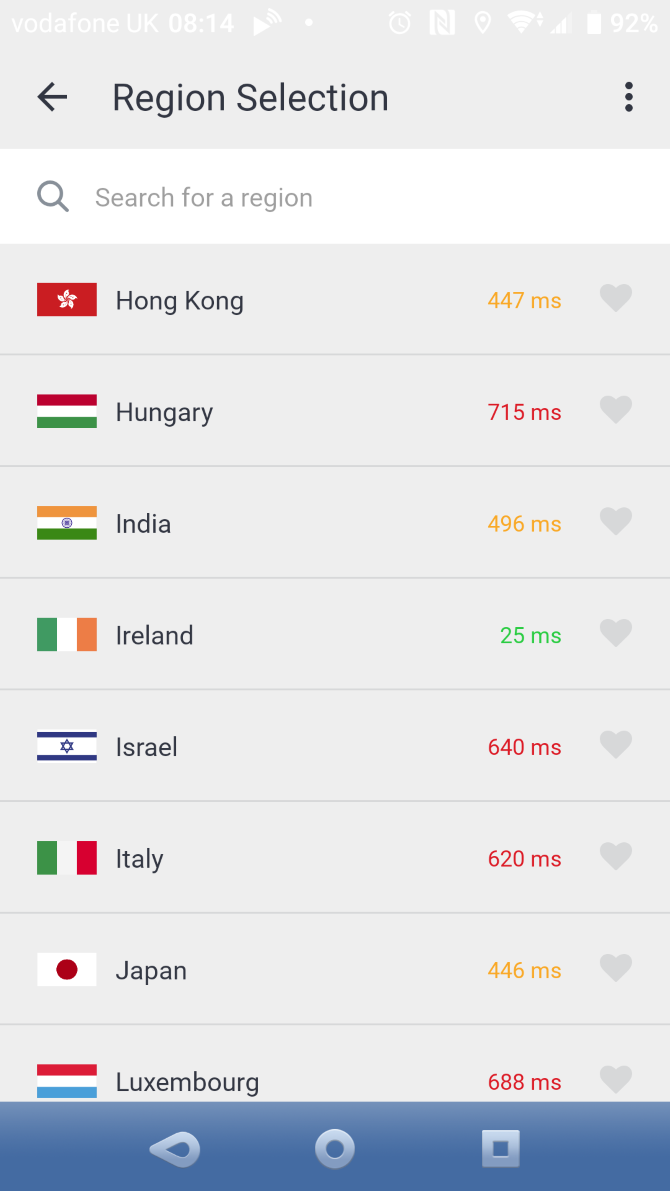In the image, there is a light blue background with a section of white text at the very top, which is unfortunately unreadable. To the left, a black arrow labeled "Region Selection" points to a smaller text area with three dots indicating more options. Below this area, there is a white rectangular search box featuring a magnifying glass icon and the prompt "Search for a region."

The main part of the image showcases a list of countries set against the blue background, each accompanied by a flag and a corresponding latency measurement in milliseconds (MS). Detailed information for each country is provided as follows:

- Hong Kong is depicted with a red flag adorned with a white star, marked at 447 MS and followed by a diamond or heart shape.
- Hungary features a flag of horizontal red, white, and green stripes, showing a latency of 715 MS and a heart icon.
- India's flag comprises orange, white, and green horizontal stripes with a blue wheel (Ashoka Chakra) in the middle, denoting 496 MS and a blue heart icon.
- Ireland is represented by vertical stripes of green, white, and orange, with a latency of 25 MS and a heart icon.
- Israel's flag, white with two blue horizontal stripes and a blue Star of David in the center, records a latency of 640 MS and a heart icon.
- Italy's flag displays vertical stripes of green, white, and red, showing a latency of 620 MS and a heart icon.
- Japan has a simple flag with a white background and a central red circle (the Sun), displaying a latency of 446 MS and a heart icon.
- Luxembourg's flag features horizontal stripes of red, white, and blue, marked at 688 MS and accompanied by a blue heart icon.

At the bottom of the image is a blue box containing three symbols: a left-pointing teardrop shape, a circle, and a square. These elements likely represent additional options or actions.

Overall, the image appears to be a user interface for selecting a region based on network latency, complete with search functionality and visual representations of latency data for various countries.